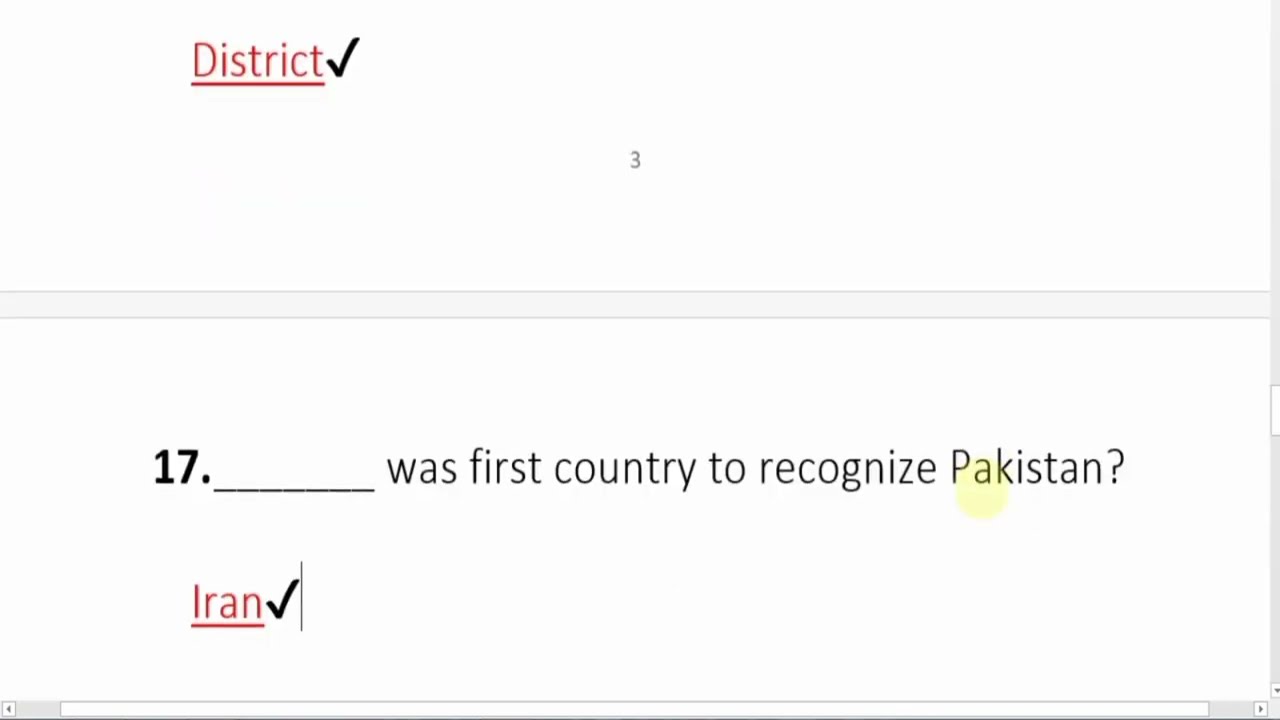The image depicts a computer screen displaying two sections of a webpage, potentially from an online exam or educational software. The background color is predominantly light gray. At the top, there's a rectangular block labeled 'district' in red, underlined, with a black checkmark next to it. In the center of this block, '3' is printed in black, indicating the page number. Below this block is another rectangular section featuring the bold number '17' with a dot underneath it, followed by a black horizontal line. The text asks, "was first country to recognize Pakistan?" The word 'Iran' in red print is beneath the question, also accompanied by a black checkmark. A slider bar is visible on the right side of the screen, suggesting that the page can be scrolled to reveal more content. This structured layout and visual cues indicate the context of the image as part of an online exam interface.